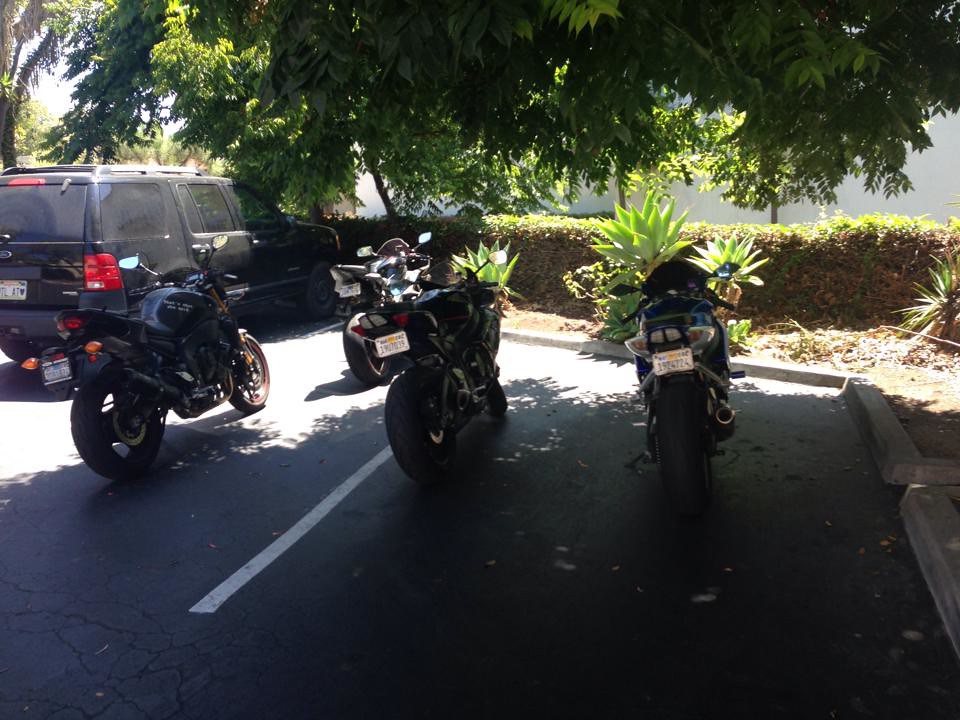The daytime photograph captures a shaded parking lot beneath a low-hanging, dark green tree that provides cover for most of the vehicles. The lot features four motorcycles, with three parked closely together within a single white-lined parking spot, and another positioned slightly away in shade. Adjacent to the motorcycles is a large black SUV, partially illuminated by sunlight; its back end glows in the sun while the hood remains shaded. The SUV's license plate reads "TL AT" with a heart symbol. The parking lot is bordered by a line of hedgerows, light green on top but browning towards the back, possibly due to lack of sunlight or winter damage. In the foreground, vibrant, spiky-leaved plants, resembling hostas or possibly yuccas, add vivid greenery. The background showcases trees with thick foliage contributing to the overall dappled shade. The entire scene illustrates a juxtaposition of sunlit and shaded areas, making for a stark contrast against the dark asphalt, highlighting the tranquil, leafy setting of this parking lot.